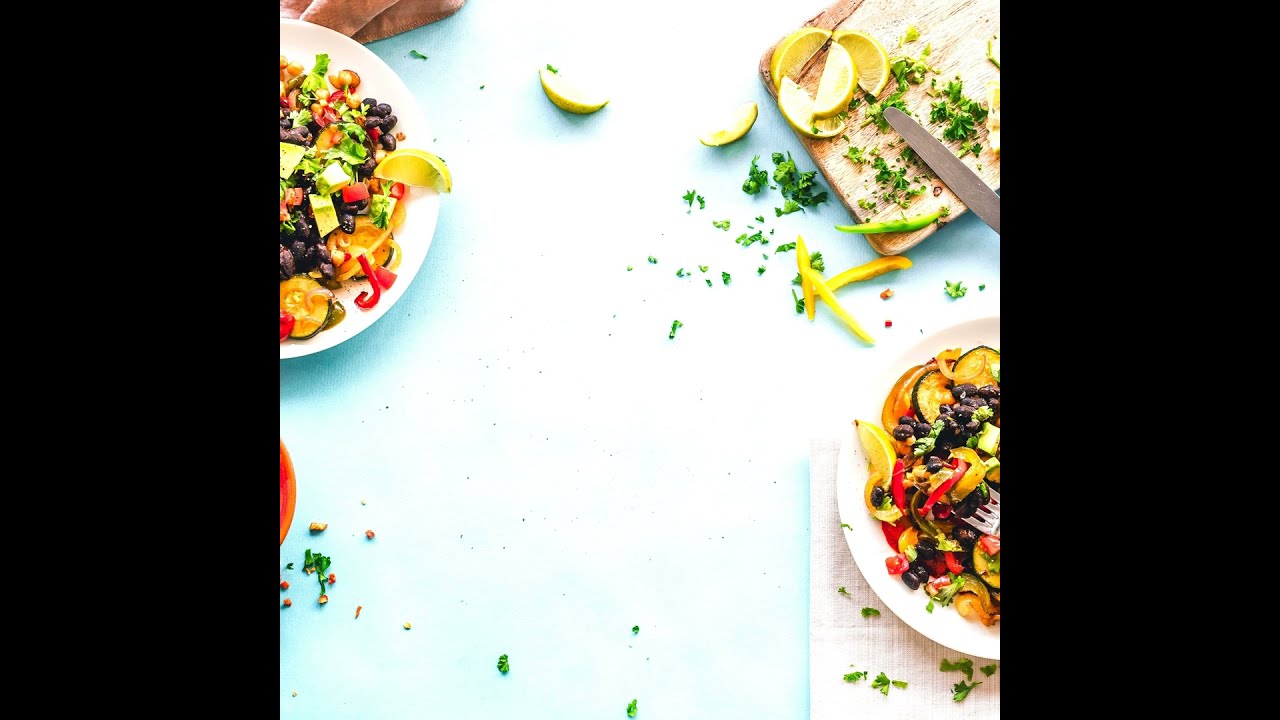The image features a vibrant, well-arranged assortment of food on what appears to be a blue tablecloth, possibly set indoors in a kitchen or restaurant. The main focus is on three white plates, each partially visible, positioned in the upper left, upper right, and bottom right corners. These plates are adorned with a colorful array of food items, including black beans, yellow lemon slices, chopped cucumbers, orange and red peppers, chunks of avocado, and sprigs of parsley or cilantro. 

Additionally, there are loose green leaves and vegetable pieces scattered across the tablecloth. In the upper right, a wooden cutting board holds several sliced lemons and limes, alongside green and yellow bell pepper slices, and a knife. A hand is seen towards the top left, possibly arranging or preparing the food. The background is completely black, highlighting the vibrant colors of the food. This image, devoid of any text, appears to be designed as a background for additional content.